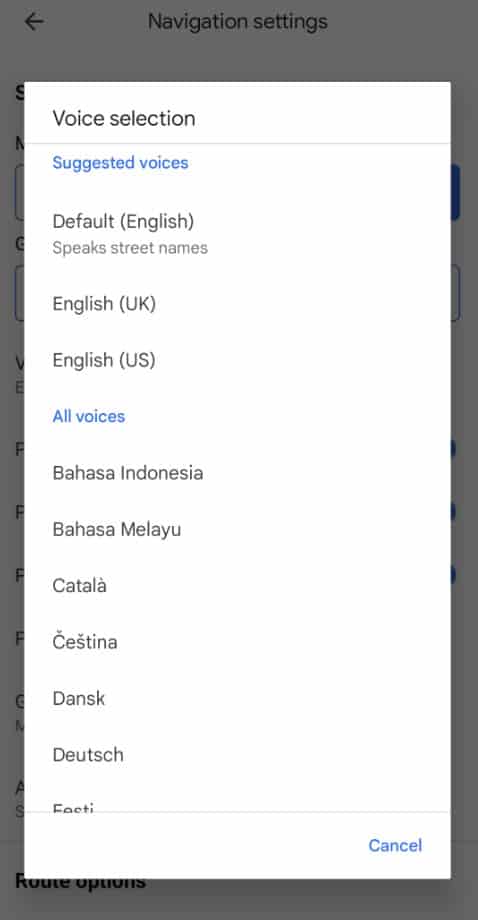The image in question is a screenshot taken from a mobile phone's screen, showcasing the navigation settings of a particular application. The background of the screen is predominantly gray. At the center is a white pop-up rectangle titled "Voice Selection." Directly underneath the title is a faint gray line, followed by the label "Suggested Voices" in clickable blue text.

Further down, the screen displays several options for voice navigation. The first option is "Default (English)" with a checkbox indicating that it includes the feature to "Speak street names." Subsequently, the list includes various English dialects, specifically "English (UK)" and "English (US)." 

Below these English options, another clickable blue label, "All Voices," is displayed. The list then continues in alphabetical order, starting with "Bahasa Indonesia," followed by "Bahasa Melayu," "Catalan," "Czech," "Danish," and "Dutch," among others. The list ends at the bottom with another faint gray line.

In the top right corner of the white rectangle, the option to "Cancel" is present in bold blue letters, indicating that it is a selectable button.